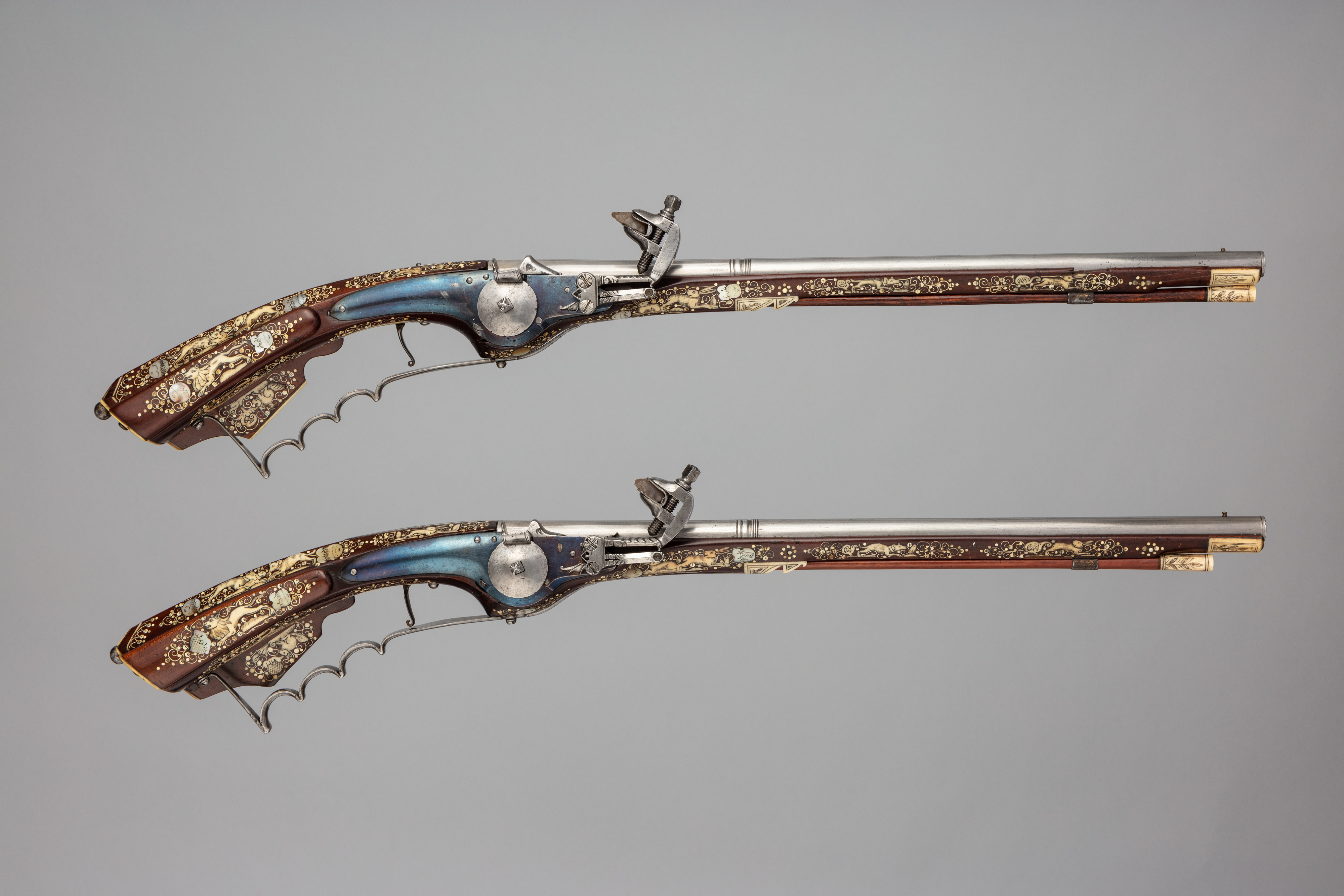This professionally captured, square photograph showcases two identical, antique flintlock pistols set against a gradient gray background that is lighter on the left. The pistols are meticulously crafted and presented one atop the other, highlighting their intricate details. Each pistol has a long silver barrel and a decorated trigger mechanism encased in blue and silver metal. The handles are adorned with ornate golden designs and floral patterns, extending to the brown stocks. The stocks themselves feature elegant gold prints, enhancing their vintage allure. The central areas of the pistols include blue-hued metal components, accented with silver circular fixtures integral to the trigger and firing mechanisms. These elements combine to illustrate the exquisite craftsmanship of firearms used during the British and Portuguese eras.